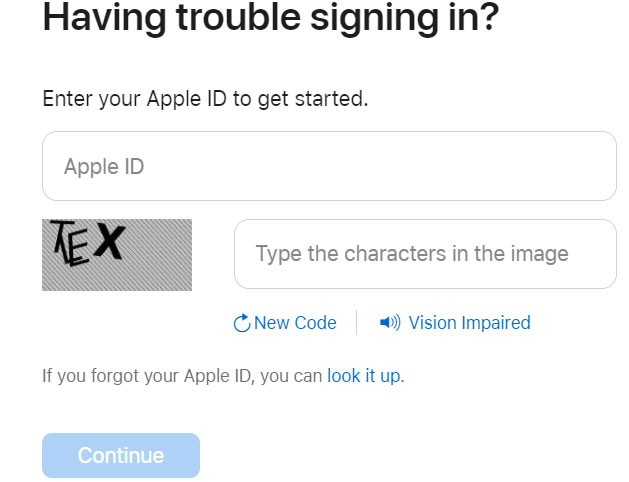The image features a user interface for an Apple ID sign-in page with a white background. At the top, black text boldly states "Having trouble signing in?". Beneath this is a white empty space, followed by smaller, non-bold black text that reads "Enter your Apple ID to get started." 

Below that, there's a rectangular input box with rounded edges labeled "Apple ID." Directly underneath it, a gray box displays a CAPTCHA with the letters "T-L-E-X." Adjacent to the CAPTCHA, another rectangular box with rounded edges prompts users with grey text that says, "Type the characters in the image."

To the right of the CAPTCHA, there is a blue hyperlink labeled "New code" for refreshing the CAPTCHA. Next to this hyperlink, a sound icon appears with the text "Vision impaired," likely indicating audio assistance. Further down, gray text suggests, "If you forgot your Apple ID you can look it up," with "look it up" presented as a blue hyperlink.

At the bottom left corner, a blue rectangular button with white text inside reads "Continue."